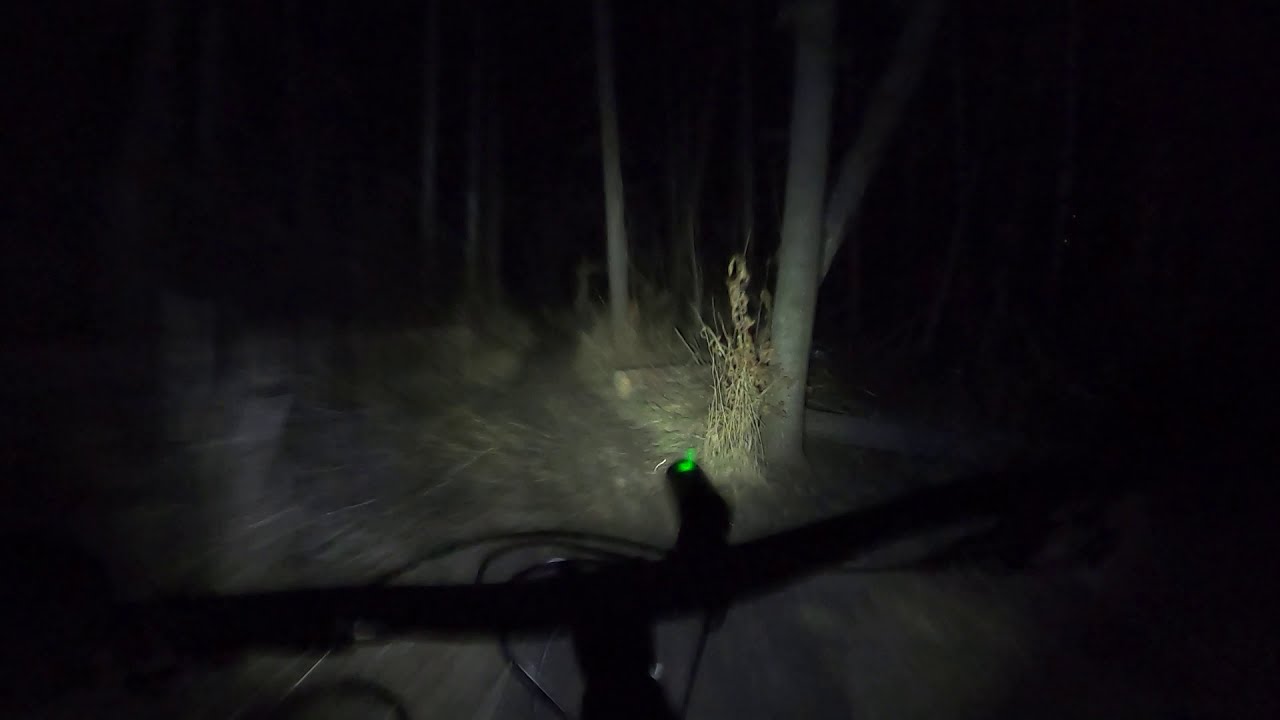The image captures a nighttime scene in a forest, shrouded in darkness. The photograph is horizontally aligned and quite blurry, suggesting movement. At the bottom center of the image, the black handlebars of a mountain bike are visible, adorned with brake wires. A bright green light, presumably a bike light, emanates from the handlebars, casting its glow on the surroundings. This light partially illuminates a narrow dirt path flanked by thin, vertical tree trunks of a light brownish-gray hue and clusters of dead grass or shrubs. The top portion of the image fades into complete blackness, adding a sense of eerie solitude to this nocturnal woodland scene. The overall setting is that of a cyclist navigating through a dense, dimly-lit forest path at night.